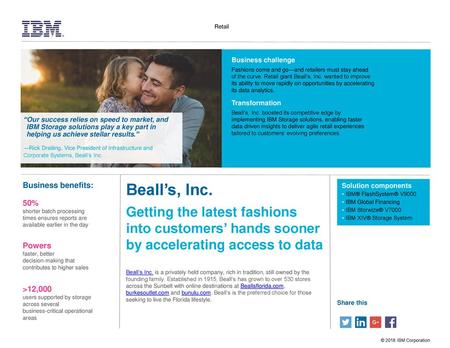**Caption:**

The website page features a blue backdrop with a prominent IBM logo in black in the upper left-hand corner, characterized by white lines that traverse it. Centrally positioned is the blurred word "recall" in black, underlined by a thin gray line. Below this, to the left, is a heartwarming image: a Caucasian toddler with blonde hair wearing a white dress adorned with blue flowers is seen kissing the cheek of a gentleman with dark hair, clad in a blue shirt. 

Beneath the photo sits a caption in blue that reads, "Our success relies on speed, biomarket," followed by, "and IBM storage solutions play a key part," and then, "helping us achieve stellar results." Below this in bluish-green text, it is signed off with a dash followed by "Rick Donning, vice president of..." though the text becomes unclear. 

On the right side of the image, inside a blue box, the heading "Business challenges" appears in white at the upper left, followed by four rows of blurred black text. Below it, "Transformation" is written in white with another four rows of blurred black text beneath. 

Further down, under the blue heading "Business benefits," the red text "50%" is visible, pointing to "Shorter batch processing" in black. Below this, two additional blurry text rows lead to the word "Powers" highlighted in red, followed by three clouded lines of text. An arrow pointing right and the red text "12,000" appear before another unclear block of four black text rows. 

In the bottom center of the page, "Beals' Inc." is printed in blue, followed by the teal statement, "Getting the latest fashions into customers' hands sooner by accelerating access to data." Five lines of text follow, interspersed with four blue, underlined words that unfortunately blur into the background.

Adjacent to this, another blue box contains the title "Solution Component" in white, succeeded by a list of four items marked with white dots, though the details remain indistinct due to blurriness. The bottom right corner features "Share this" in blue, next to a blue Twitter icon (a white bird in a blue box), a LinkedIn icon (blue box with white "IN"), an orange box whose contents are unclear, and a blue box with a white lowercase "f" symbol for Facebook.